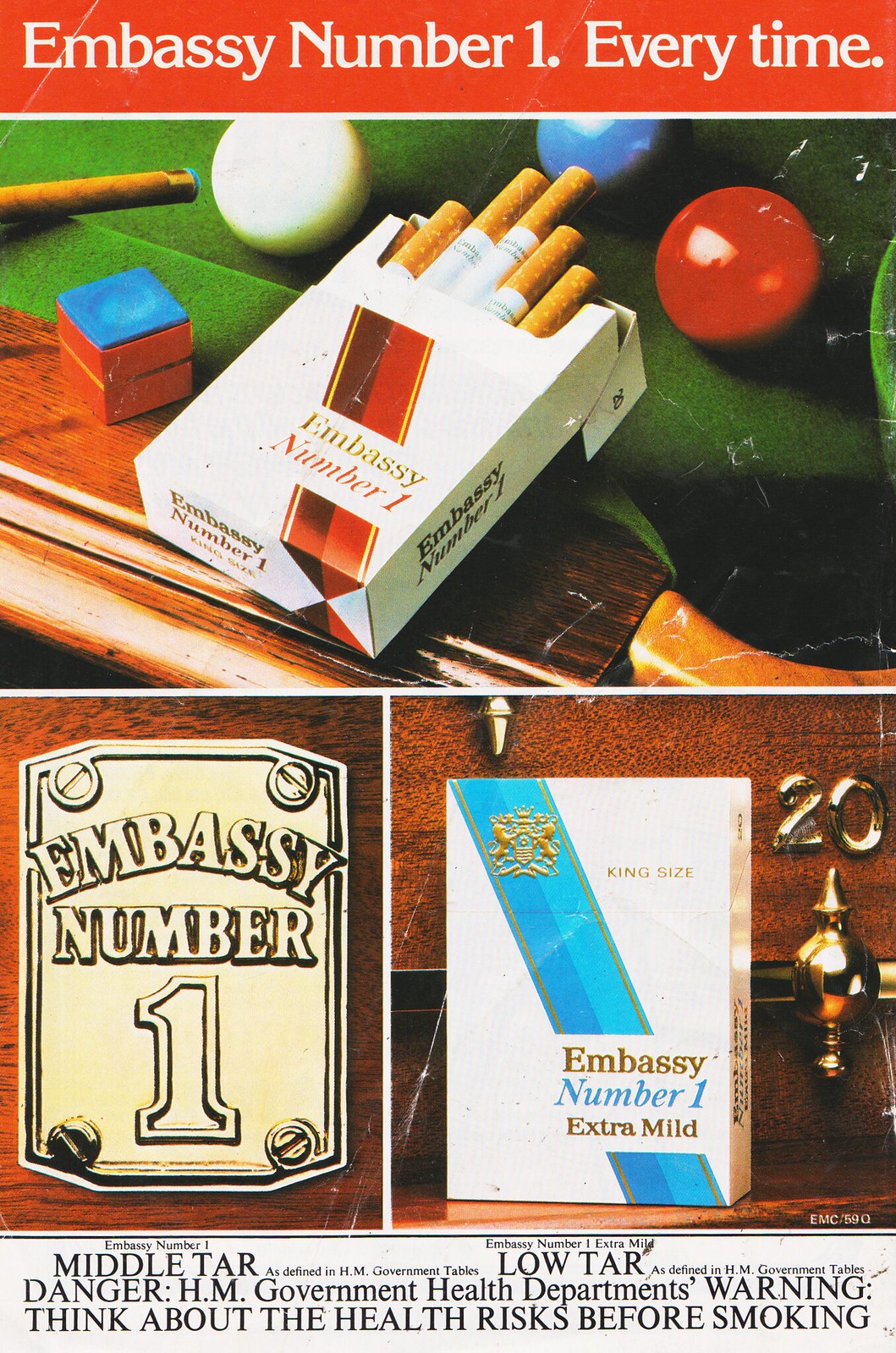This advertisement for Embassy Number 1 cigarettes is a color image divided into three sections. At the top, a bold red bar with white text states "Embassy Number 1 every time." Below this, the top half of the image features a photo of an open white carton of Embassy Number 1 cigarettes, identifiable by a red stripe on the carton. The cigarettes, which are filtered, are protruding from the open carton, positioned on the green felt surface of a pool table. Accompanying this is a visual of pool paraphernalia, including a white, blue, and red ball near the corner pocket, a piece of blue chalk, and the end of a pool cue with a blue tip.

The bottom half of the advertisement is split into two images. On the left, a shiny brass-colored decal with the text "Embassy Number 1" appears as though placed on wood. On the right, there's a box of King Size Embassy Number 1 Extra Mild cigarettes, distinguished by a blue diagonal stripe and a gold number 20. At the very bottom, black text on a white background warns, "Embassy Number 1 Middle Tar, Embassy Number 1 Extra Mild Low Tar. Danger. HM Government Health Department's Warning: Think About the Health Risk Before Smoking."